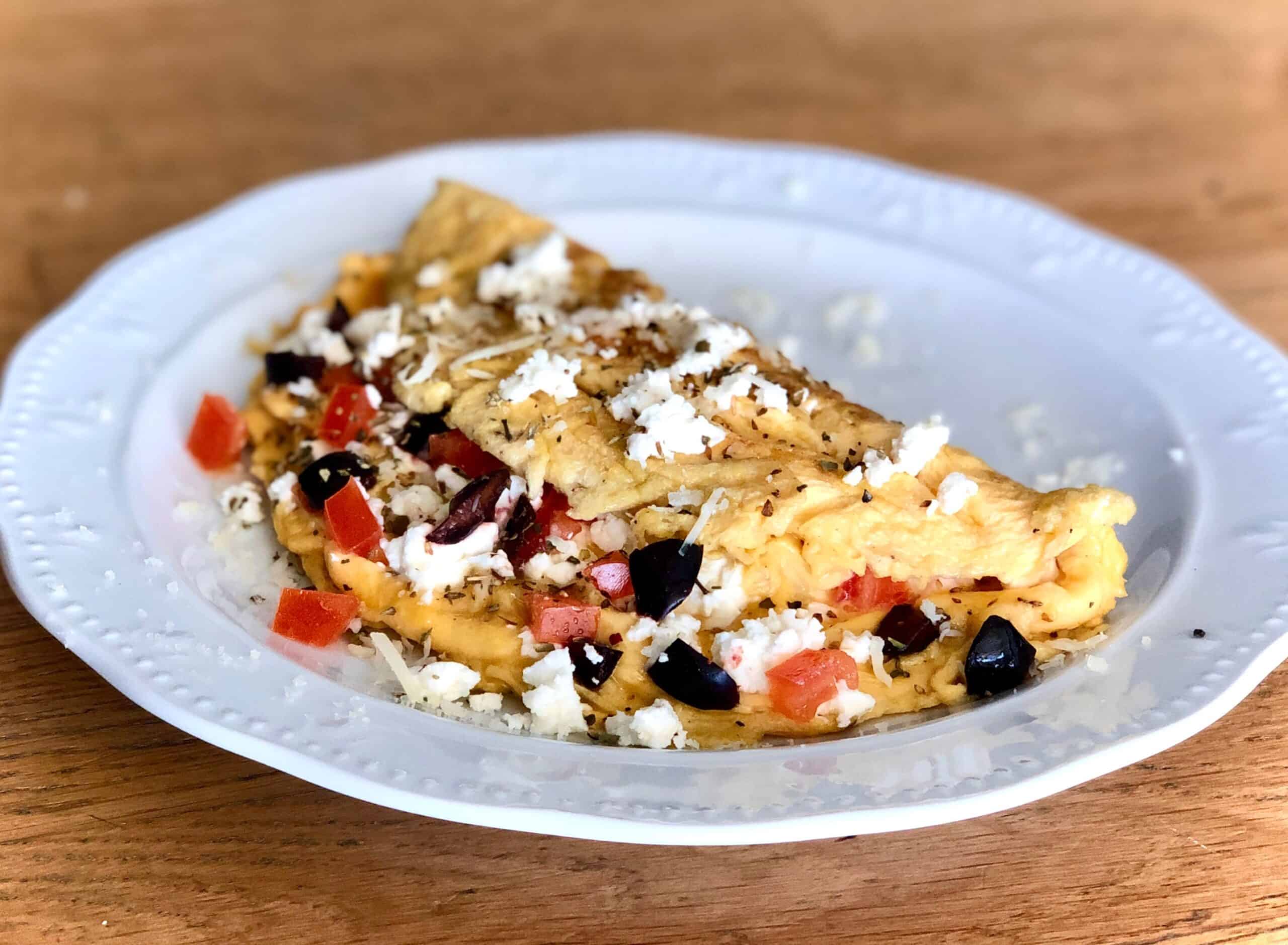The image features a visually appealing omelet on a decorative white plate, centered on a light brown wood table with a visible grain. The omelet, primarily yellow, is folded and contains vibrant ingredients including red tomato slices, black olives, and maroon chili peppers, all interspersed with melted cheese. Additional cheese is sprinkled on top, adding a whitish accent to the dish. The surrounding plate is mostly visible with the wood table forming the background, notably exposed in the corners of the image. The clear, detailed arrangement and vivid colors make this image ideal for use in a recipe website or culinary presentation.